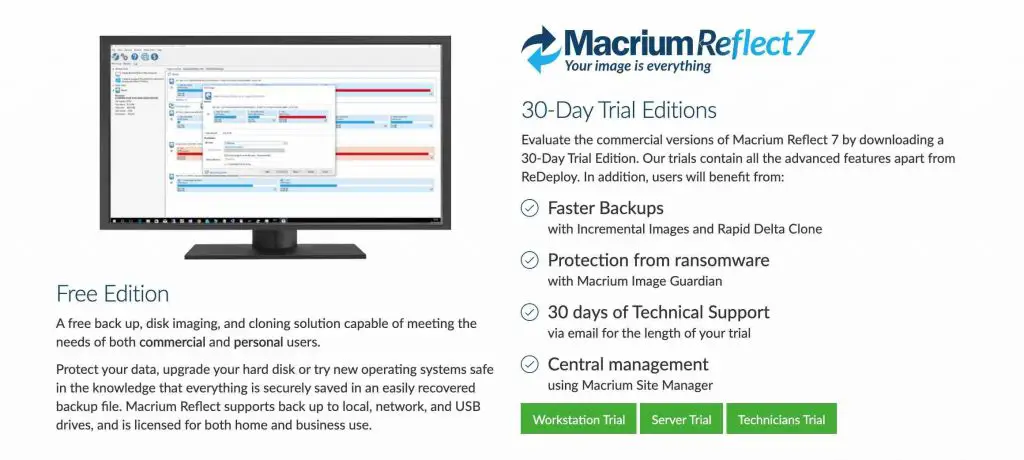**Detailed Caption:**

This image is a screenshot showcasing Macrium Reflect 7, a prominent data backup, disk imaging, and cloning solution. The logo is prominently featured at the top left, consisting of two interlocking arrows—one darker blue and one lighter blue—accompanied by the text "Reflect7" in a lighter blue font to the right of the logo. Below the logo, the text states "Free Edition. Free backup, disk imaging, cloning solution capable of meeting the needs of both commercial and personal users," highlighting the versatility of the software.

In the center of the image, there's a wide desktop computer screen displaying various bar graphs and windows, indicating the software's user interface. On the right side of the image, under the logo, it is mentioned that Macrium Reflect 7 offers a "30-day trial edition," allowing users to evaluate the commercial version. The trial includes almost all advanced features except for Redeploy and provides four significant benefits outlined with check marks: faster backups, protection from ransomware through Macrium Image Guardian, 30 days of technical support, and central management with Macrium Site Manager.

Additionally, the image promotes the trial options with three buttons labeled "Workstation Trial," "Server Trial," and "Technicians Trial," encouraging users to download and experience the comprehensive capabilities of Macrium Reflect 7 for a 30-day period.